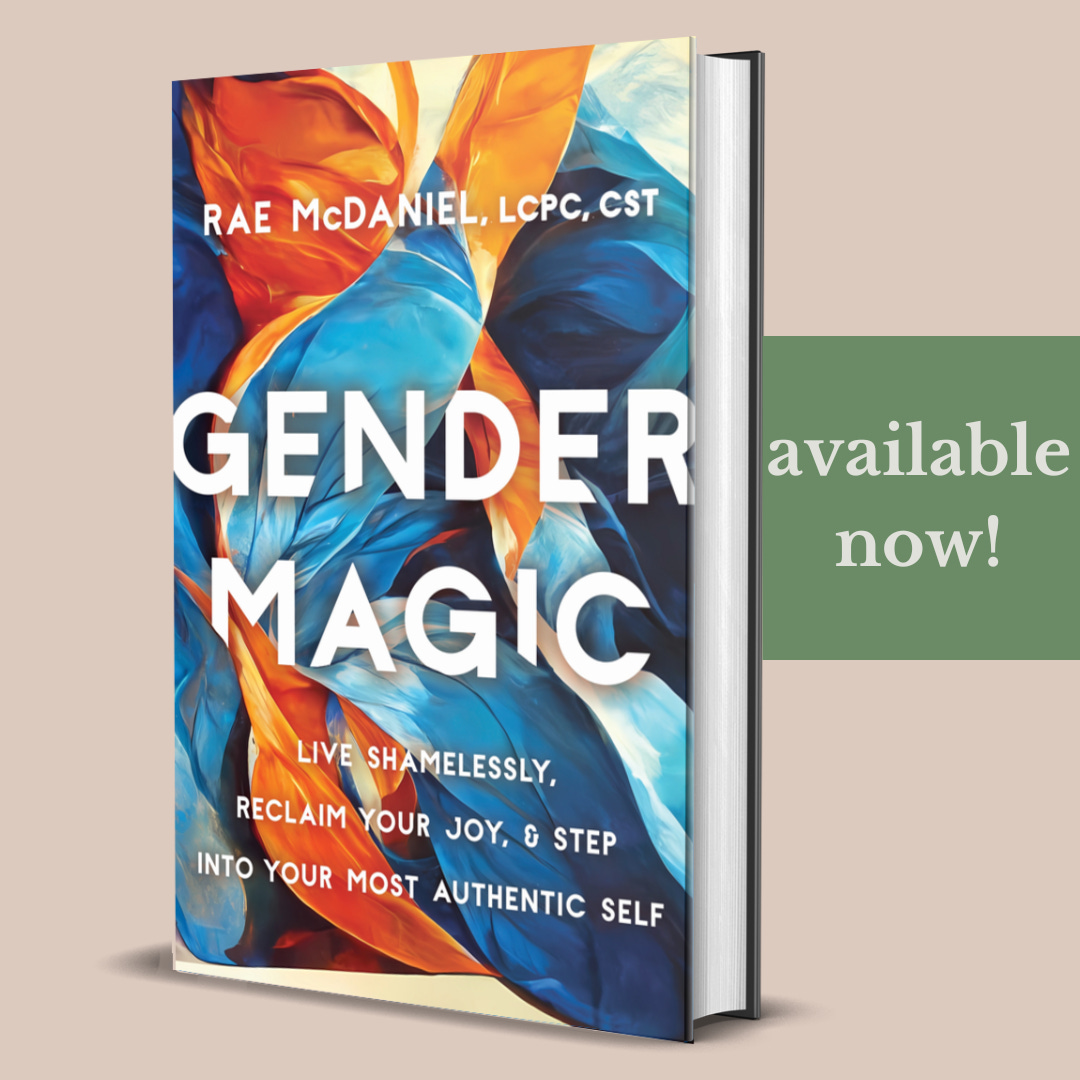This graphic features a promotional image of a book against a beige background. Central to the image is the book, which is slightly angled to the left, displaying part of its page side on the right. The vibrant cover art resembles a dynamic, wavy fabric or an abstract oil painting with splashes of blue, orange, dark blue, light blue, and red hues. Bold white text stands out against this colorful backdrop, starting with the author's name at the top: Ray McDaniel, LCPC, CST. Dominating the center of the cover, large white letters spell out the title: "Gender Magic," partially integrated with the artwork and featuring a subtle drop shadow or gray outer glow. Below the title, an inspiring tagline reads: "Live Shamelessly, Reclaim Your Joy, Step Into Your Most Authentic Self." To the right of the book, a green rectangular text box with white font announces, "Available Now!"